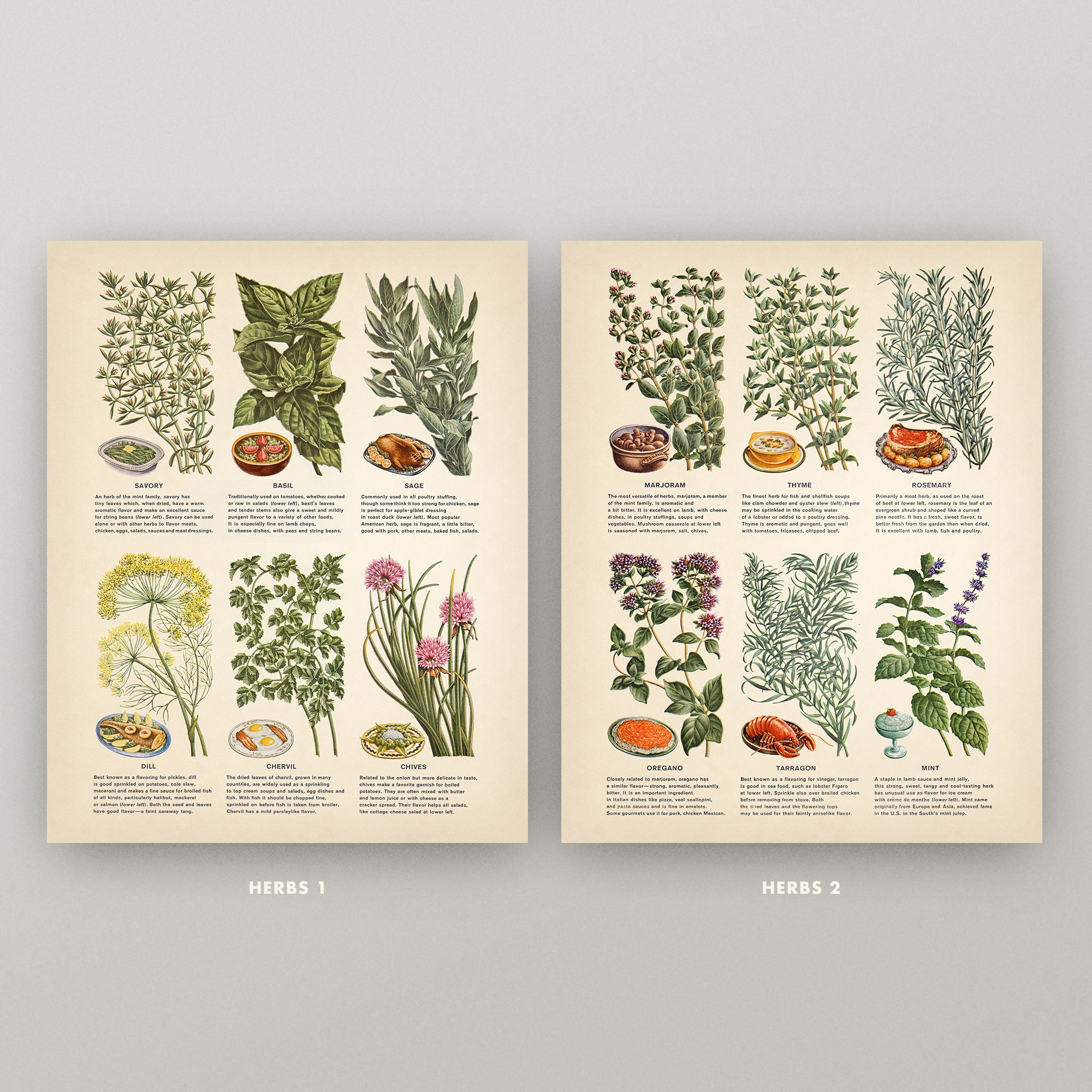The image features two pieces of paper, possibly book pages or posters, set against a gray background. Each page showcases six different types of herbs, each with detailed illustrations and small descriptions below them.

The first page, labeled "Herbs 1," includes six herbs. From the top left:
1. A herb with thin leaves, depicted in a container of green leaves.
2. Another herb with very large, dark green leaves marked by black lines.
3. A herb with erect, light gray leaves.
4. One with stems crowned by a tuft of yellow flowers.
5. A herb with slender roots and thin green leaves.
6. Grass-like hairs topped with pink flowers.

The second page also displays six herbs, beginning in the upper left:
1. A herb with upright stems and numerous small green leaves, topped with small bulbs.
2. Another with straight green stems and leaves.
3. A herb characterized by stems with thin, grayish hairs having a blue tint.
4. One with broad green leaves and dark purple flowers at the top of the stems.
5. A herb in the middle with thin stems and leaves in various directions, illustrated with a lobster on a plate below it.
6. The last herb, in the bottom right corner, has large green leaves and a singular, straight shoot bearing purple flowers.

Each page has a yellow background that transitions from a darker shade at the top to lighter shades towards the center. The meticulous illustrations are accompanied by tiny, unreadable explanatory paragraphs under each herb.